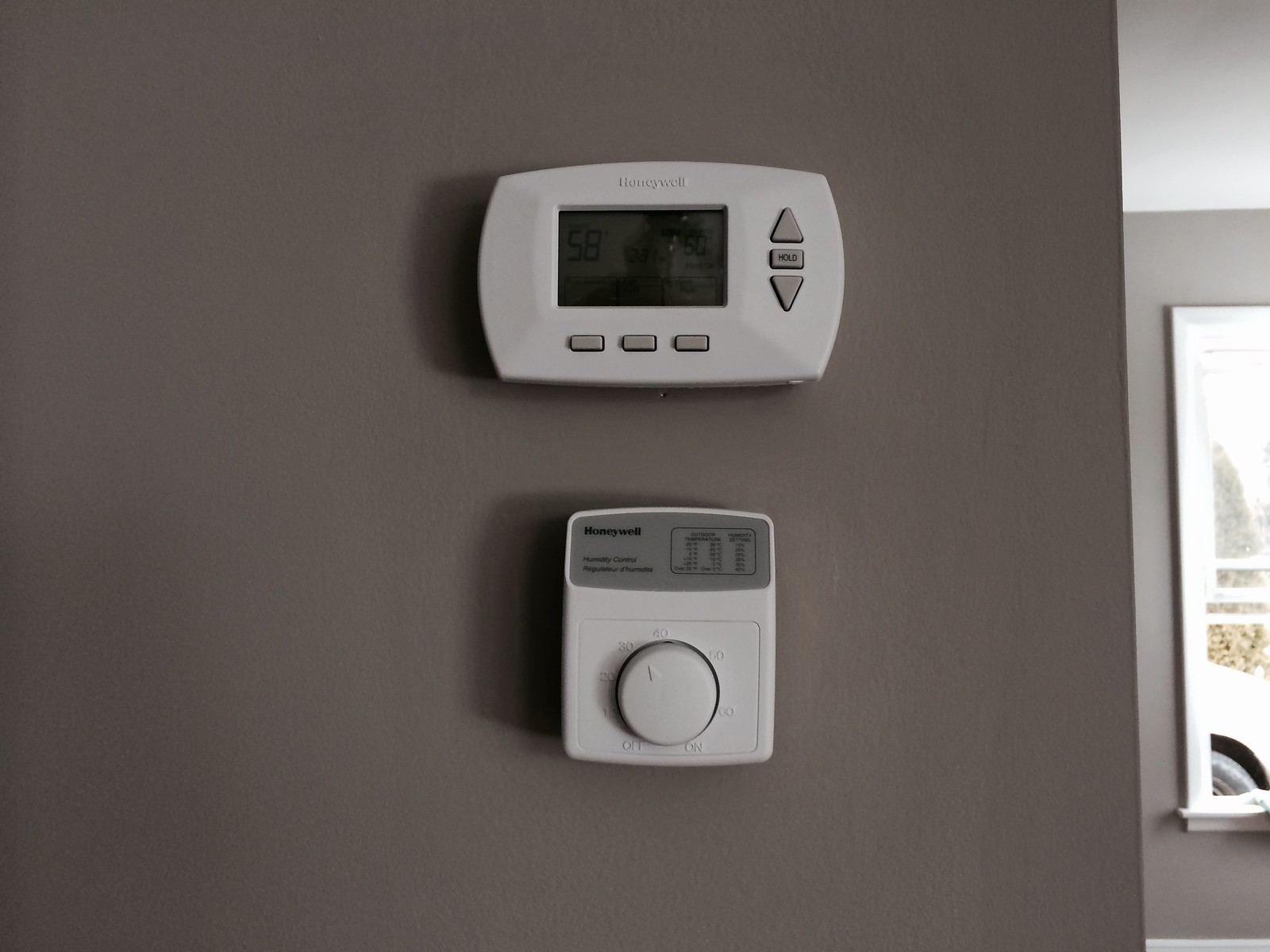This photograph showcases a white, rectangular Honeywell programmable thermostat mounted on a dark gray wall. The thermostat features easily identifiable gray buttons and displays a temperature of approximately 58 degrees. Directly below the thermostat, there is another smaller Honeywell device equipped with what seem to be power buttons, possibly functioning as a timer, although the exact details are difficult to discern due to its size.

To the side, part of a painting or photograph on a white canvas is visible. The artwork contains hints of brown and silver hues and is set against a lighter gray background compared to the wall with the Honeywell devices. The room is illuminated by a light source, and the ceiling appears light-colored, suggesting a well-lit environment. The artwork seems to rest on a ledge, hinting at a framed photograph or canvas, though the specific subject remains unclear.